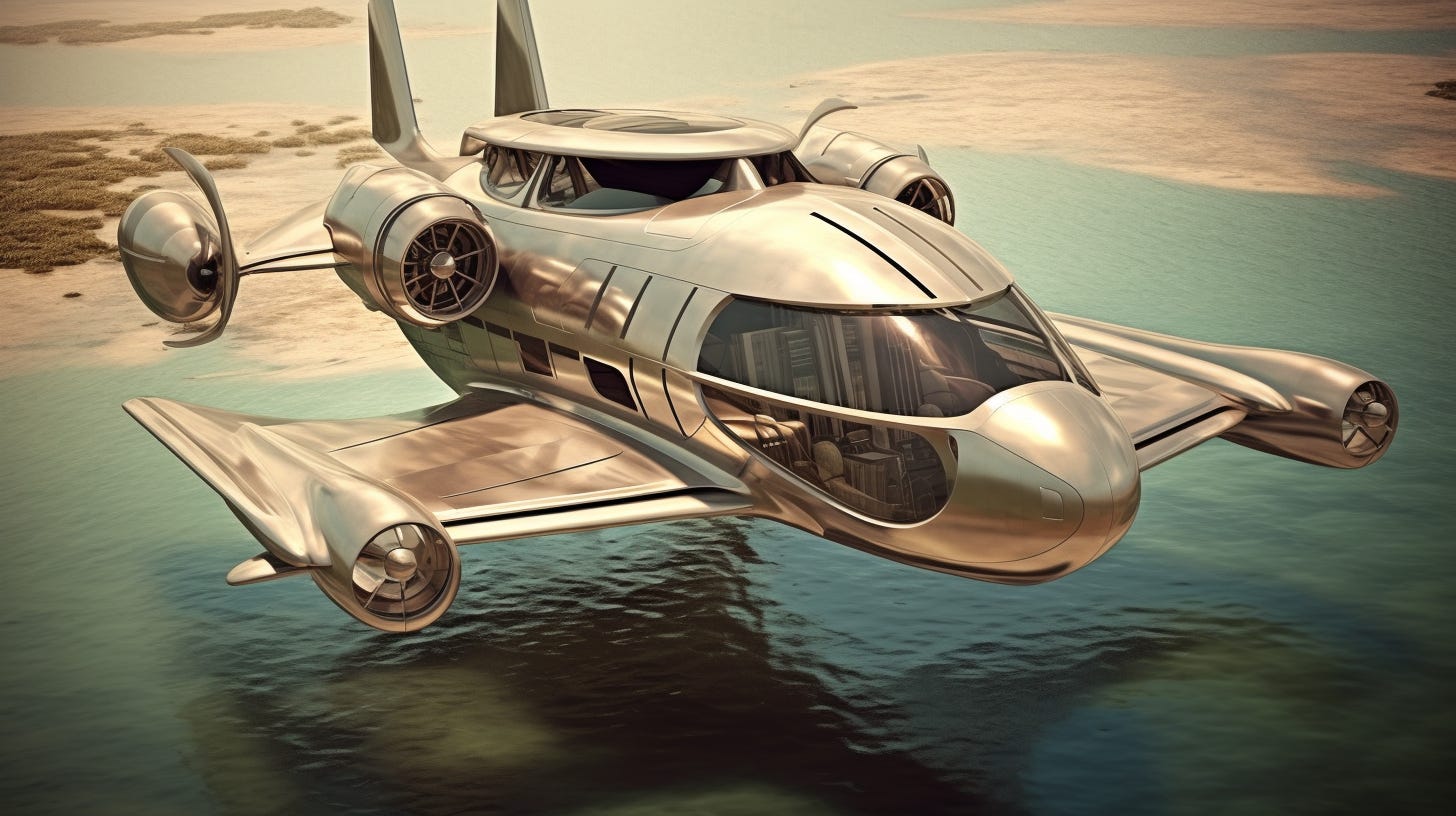This computer-rendered image depicts a luxurious starship or ultra-modern seaplane, combining deco-punk aesthetics with futuristic design. The aircraft, crafted from a gleaming gold-steel metal that reflects its surroundings, features an elongated fuselage and two prominently sleek wings. Each wing tip is equipped with advanced jet propulsion engines. The front cockpit, encased in expansive, transparent glass windows, provides a comprehensive view inside, hinting at a two-person capacity. Additionally, there's another large glass window on the side of the cockpit, enhancing visibility. Further back, near the fuselage, two more high-powered engines are positioned, likely jet or fan engines.

The scene captures the starship soaring low over a stunningly flat, green-tinged body of water, studded with small islands, accentuating a backdrop of retrofuturistic luxury. The water's reflective quality and the plane's polished surface create an array of reflections, including glimpses of the wings and possibly distant buildings. The sophisticated design evokes a blend of high society, vintage futurism, and advanced technology.